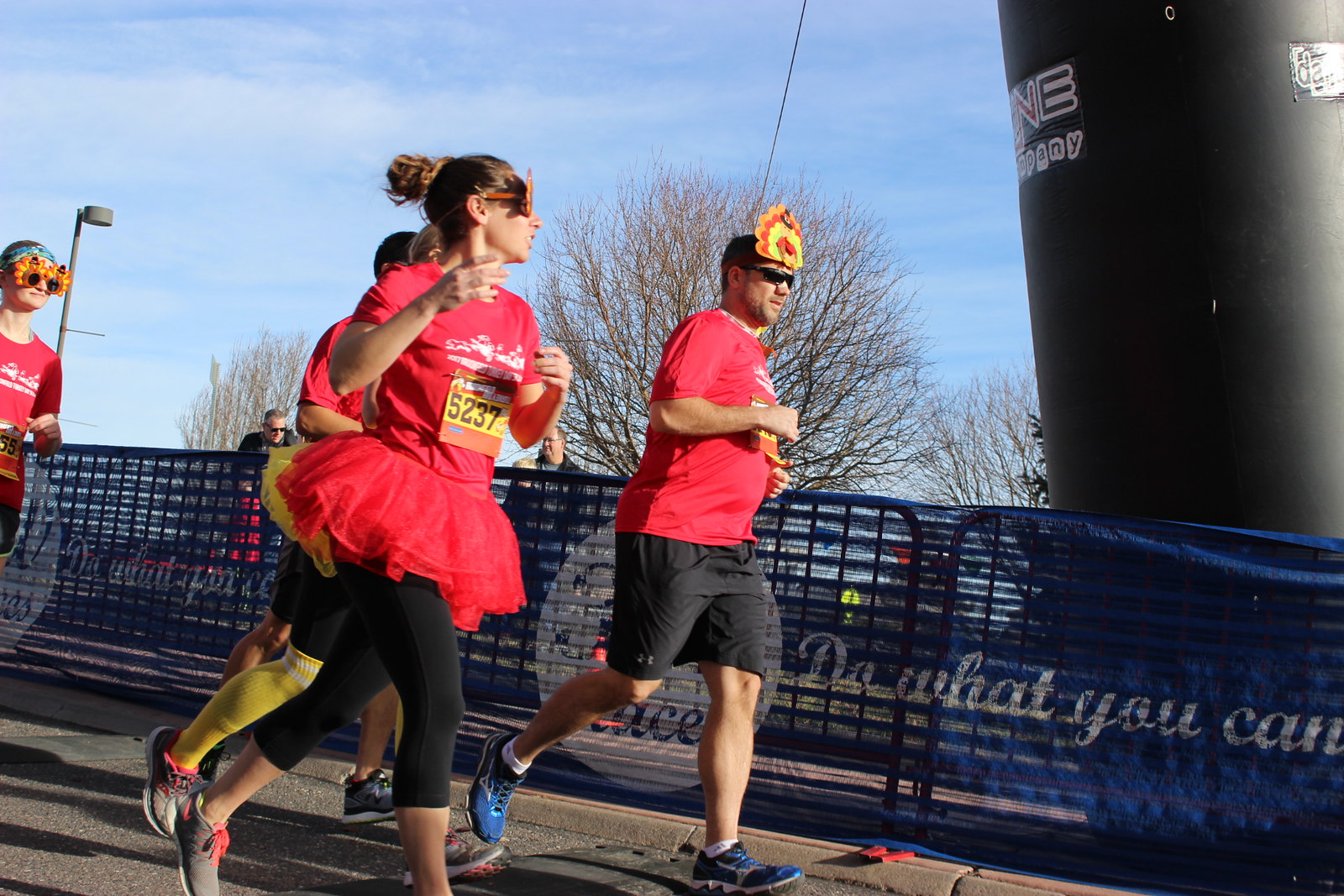The image depicts a vibrant outdoor running event on a sunny day with a clear blue sky featuring wispy clouds. Participants are dressed in festive attire, suggesting a themed race. At the forefront, a man wearing a red shirt, black shorts, blue jogging shoes, and a whimsical turkey hat stands out. Beside him, to the right, is a woman in a red shirt, red tutu, black leggings, and gray running shoes with red laces, marked with the number 5237 on her running tag. She sports turkey glasses. Behind her are two more participants: one woman adorned in a red shirt, blue bandana, and turkey glasses, and a man in a red shirt, yellow tutu, black leggings, yellow socks, and gray shoes. Another prominent figure on the left wears a red shirt, orange tutu, black leggings, oversized sunglasses, and has brown hair tied in a ponytail. A tall black pillar and a fence line the side of the road, adding structure to the racecourse. In the background, lush trees complement the cheerful atmosphere of the event.